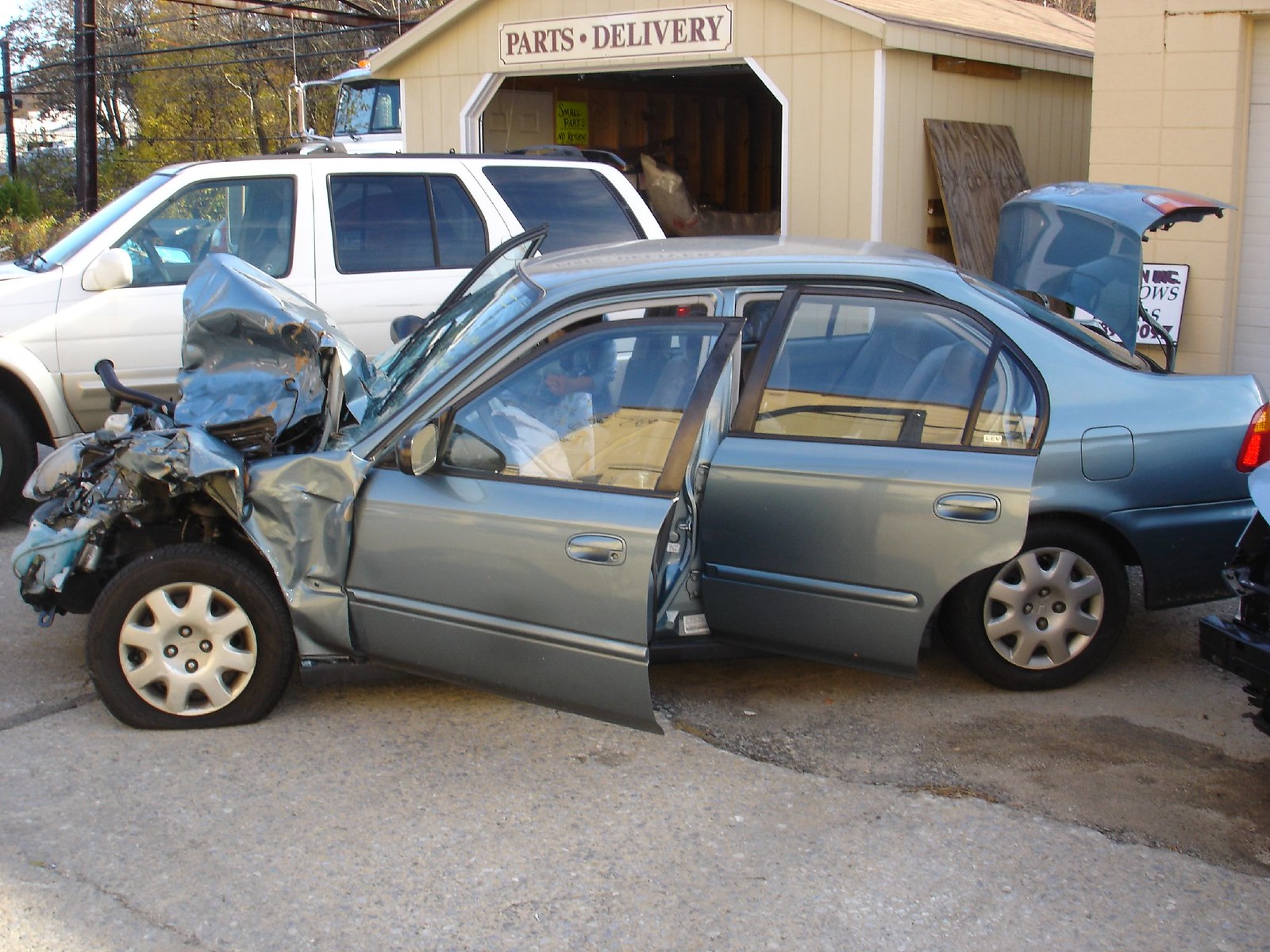The photograph captures a severely wrecked grayish-green Toyota sedan, positioned in front of a light tan garage with a sloped roof. The garage bears a sign across the top reading "parts and delivery," with several trees visible to its left. In the foreground, the damaged sedan stands out with its front end completely crumpled, missing bumper, and flat front left tire, rendering much of the engine exposed and in pieces. The driver's side is prominently displayed, showcasing open front and rear doors, as well as a deployed airbag and beige interior. Additionally, the trunk of the car is open, indicating the extent of the collision. Behind the wrecked vehicle, a white SUV with tinted rear windows is parked, appearing undamaged. A person is seen inspecting the sedan from the passenger side, adding a human element to the scene. The overall setting suggests it is a garage driveway, with a few partially visible auto parts scattered in the background, emphasizing the severity of the crash.